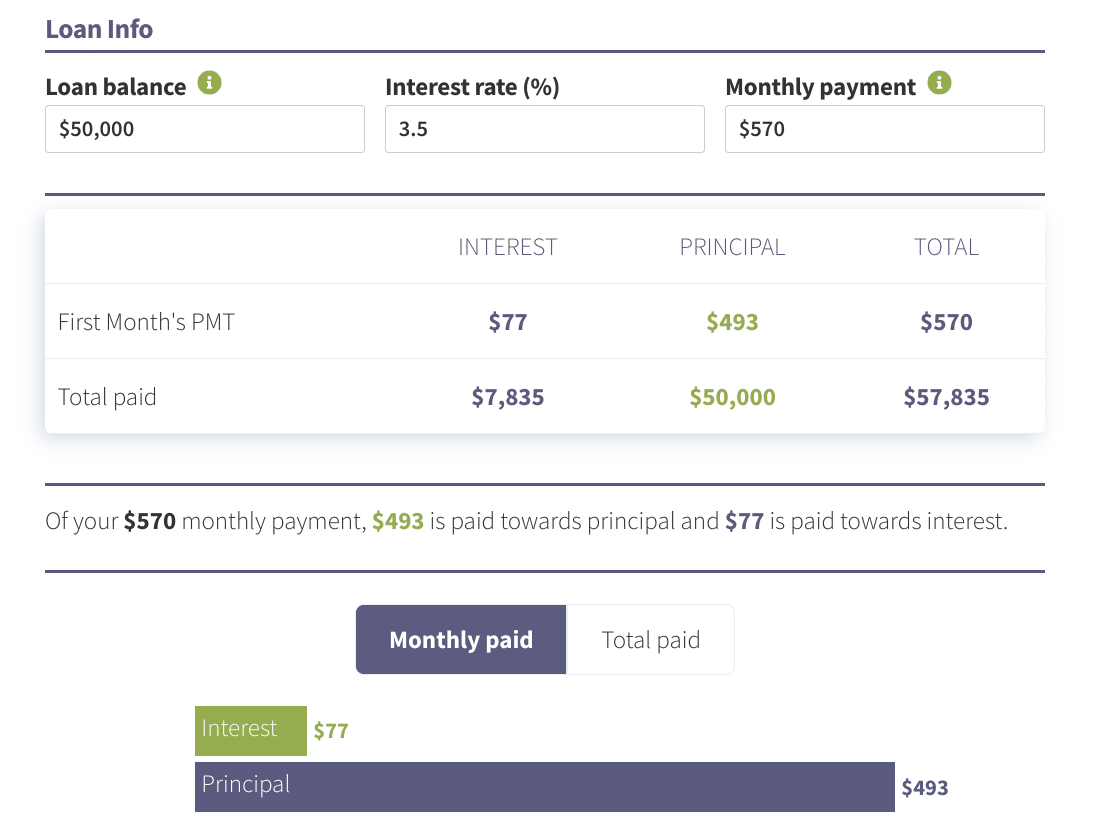The image is a detailed screenshot showcasing loan information. In the upper left corner, the title "Loan Info" is prominently displayed in purple text, separated from the subsequent content by a long horizontal bar. Below this bar, the section is organized into three main columns.

In the first column, titled "Loan Balance," a circular green icon with a white lowercase “i” is present, aligned next to the text. The displayed loan balance is $50,000. The middle column is labeled "Interest Rate," showing an interest rate of 3.5%. The rightmost column reads "Monthly Payment," indicating a monthly payment amount of $570, accompanied by another identical green icon.

Beneath this initial section, there is a line-by-line breakdown set against a white background. The first month's payment is divided into three smaller columns: "Interest," "Principal," and "Total." The interest for the first month is $77, the principal repayment is $493 (highlighted in green), and the total payment is $570 (highlighted in purple).

Further down, another section labeled "Total Paid" summarizes the overall payment details, again divided into the same three columns. The total interest paid is $7,835 (in purple), the principal amount paid remains $50,000 (in green), and the aggregate total paid is $57,835.

At the bottom of the image, additional text in black explains that from the monthly payment of $570, $493 is allocated towards the principal, and $77 goes towards interest.